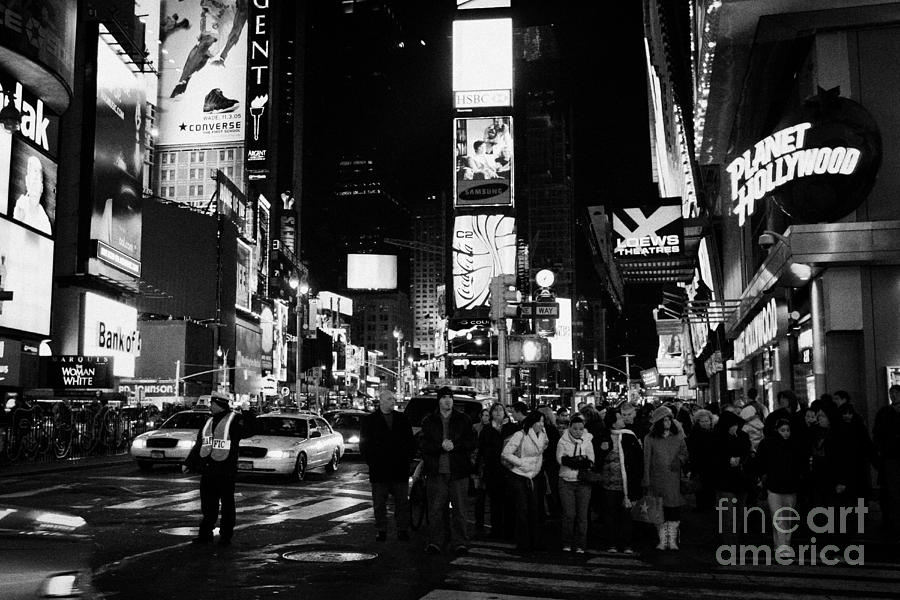This black and white photograph captures a bustling urban scene that resembles iconic cityscapes such as Times Square in New York, but it could also evoke similar areas in Los Angeles or Chicago. The image is packed with tall buildings adorned with a multitude of signs and digital panels, including distinctive advertisements for Planet Hollywood, Lowe's Theatres, Bank of America, Converse, Kodak, and Coca-Cola. The streets are alive with people bundled up in winter jackets, suggesting a cold, possibly damp, time of year. A policeman stands in the street, directing traffic amidst a flurry of yellow cabs and cars. There's a large crowd waiting at a crosswalk, adding to the overall sense of urban hustle and bustle. Notably, the Fine Art America logo is discreetly positioned in the bottom right corner of the photograph.